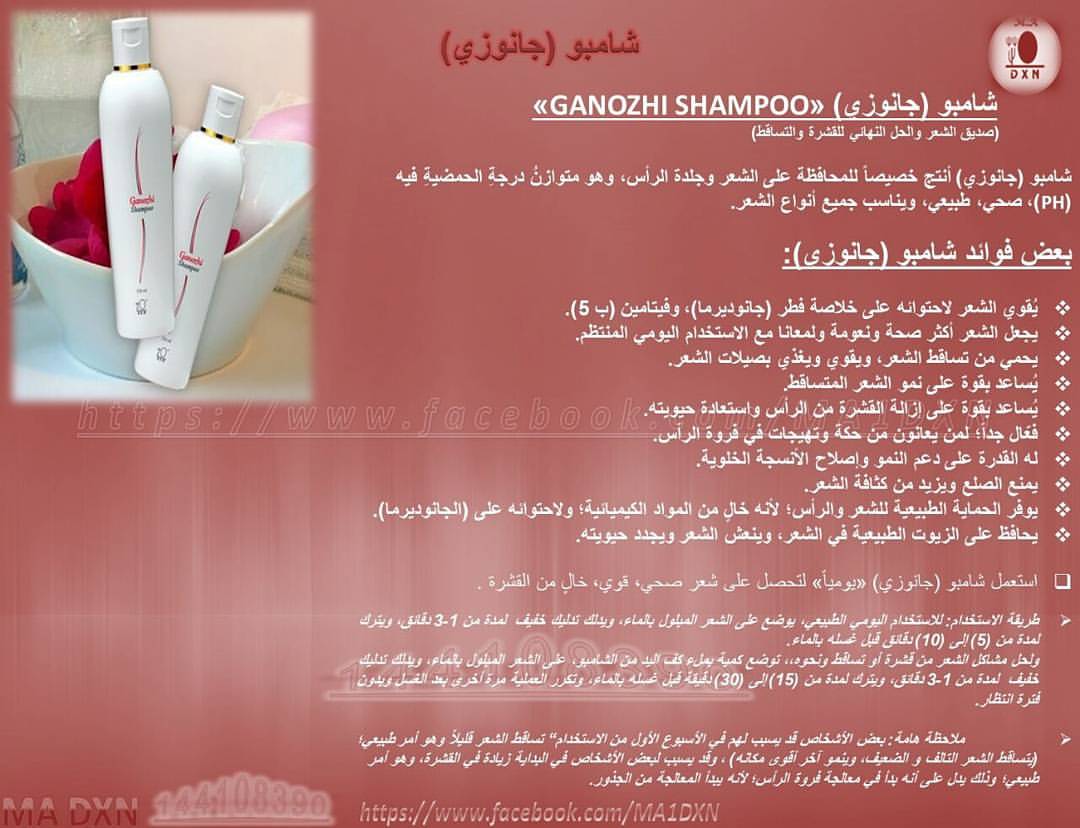The image is an advertisement for Ganozzi Shampoo, featuring a clean, peach or rose-colored background. On the top left corner, two sleek, white bottles of shampoo with gold caps are prominently displayed. These bottles are adorned with pink and black text and a distinctive curved pink line running through them. Below the brand name Ganozzi Shampoo, which is written in elegant white font at the top of the image, additional text appears in a foreign language. The ad also includes the letters "PH" and the web address "www.facebook.com/MA1DXN" at the bottom. The bottles are placed next to a blue and white wash basin filled with rose petals, situated on a pristine white surface against a white wall, adding a touch of luxury and elegance to the overall composition.